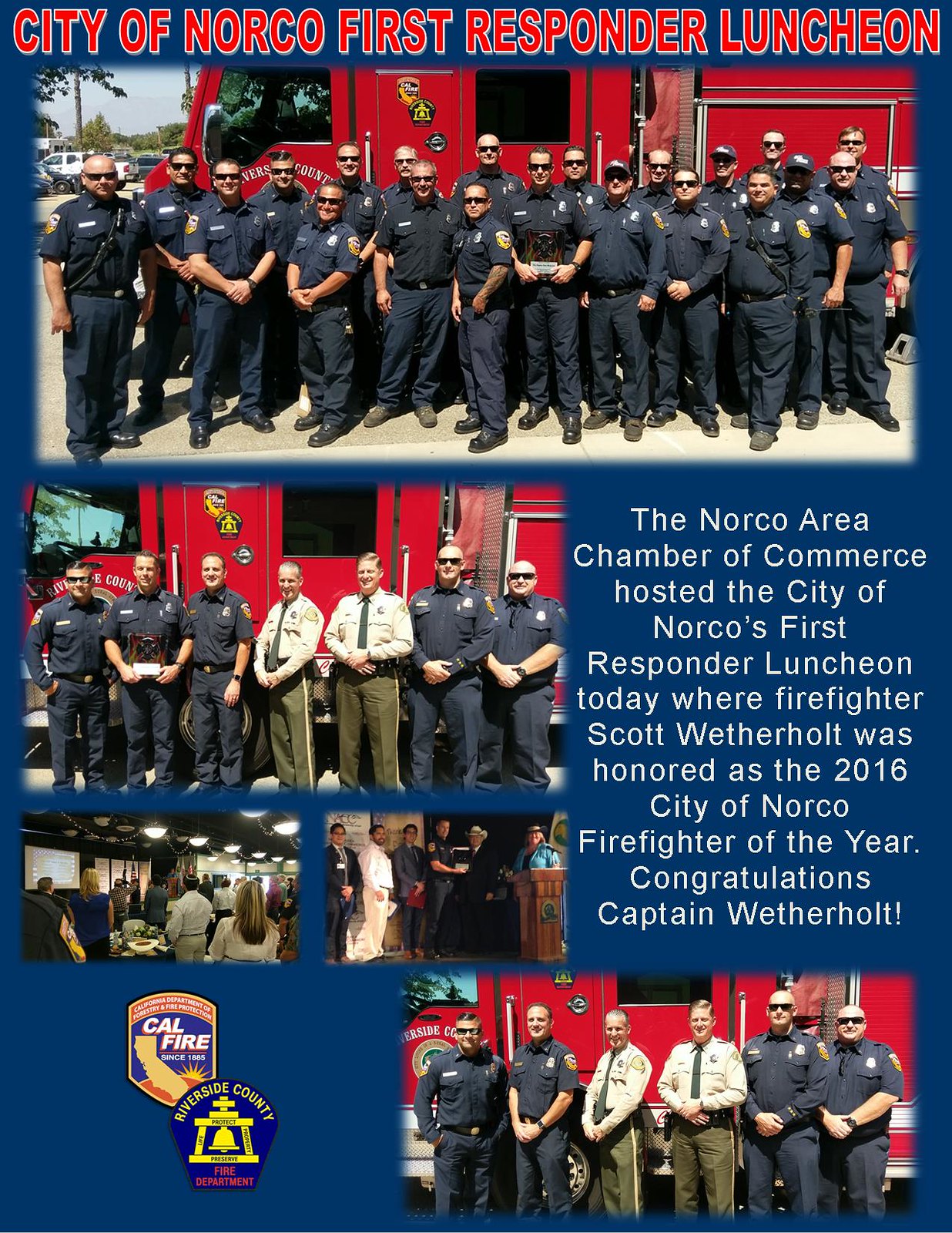The image is an advertisement for the City of Norco First Responder Luncheon, featuring a dark blue background with red text at the top that reads, "City of Norco First Responder Luncheon." Below this header is a large photograph of several firefighters in blue uniforms and sunglasses, standing in a parking lot beside a red fire truck. On the right side of the image, white text on the blue background announces, "The Norco Area Chamber of Commerce hosted the City of Norco's First Responder Luncheon today where Firefighter Scott Weatherholt was honored as the 2016 City of Norco Firefighter of the Year. Congratulations Captain Weatherholt!" 

The left side of the image contains three smaller photographs: the top one depicts more firefighters in front of a fire truck, the middle one captures people attending the luncheon, and the bottom one shows individuals next to a podium, two of whom are shaking hands, likely commemorating the event. Additionally, the CAL FIRE and Riverside County Fire Department logos are located in the lower left corner. Another photograph at the bottom right replicates the scene of firefighters posing in front of a fire truck. The overall layout honors the event while highlighting the attendees and the awards ceremony.